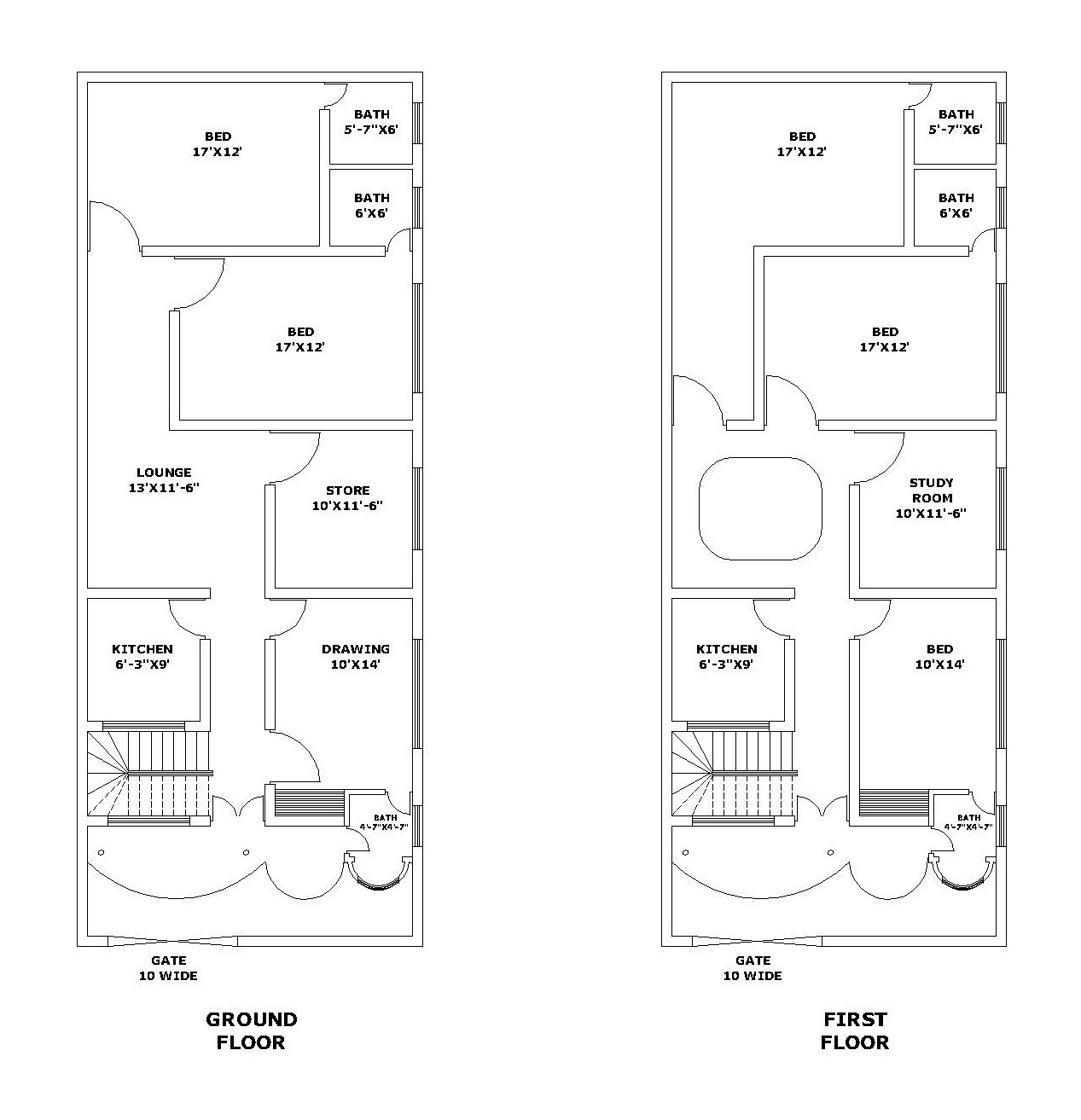This detailed architectural diagram illustrates both the ground floor and the first floor of a home. On the ground floor, the kitchen measures 6 feet by 3 feet by 9 feet and provides ample space for culinary activities. The primary bedroom is generously sized at 17 feet by 12 feet and is complemented by an en-suite bathroom that measures 5 feet by 7 feet by 6 feet. Another notable feature on this level is a lounge area, which spans 13 feet by 11 feet by 6 feet, offering a cozy space for relaxation and social gatherings. Adjacent to the lounge is a guest bathroom measuring 6 feet by 6 feet. 

The first floor features another kitchen, also sized at 6 feet by 3 feet by 9 feet, and a secondary bedroom that measures 10 feet by 14 feet. In addition, there is another bedroom on this level, measuring 17 feet by 12 feet, which mirrors the layout of the ground-floor bedrooms but may be configured slightly differently to optimize space. Notably, a staircase connects the two floors, providing easy access between levels. Overall, this home features a thoughtfully designed layout with well-sized rooms and essential amenities across both floors.